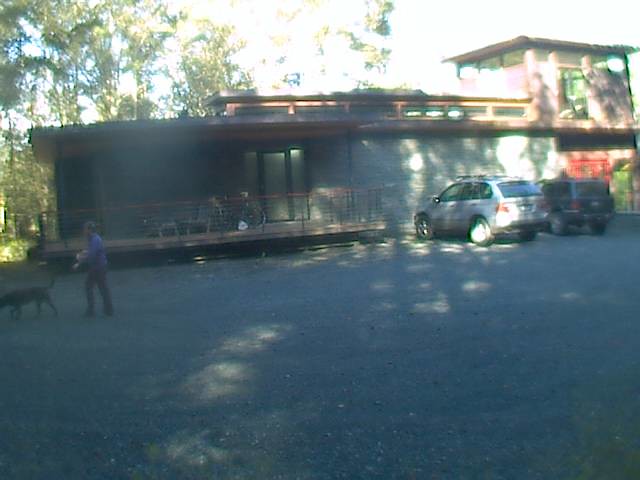In the image, there is a brick house with a welcoming porch that features two chairs and a table, suggesting a cozy spot for relaxation. The porch also has a bicycle propped up against the building. In front of the house, two vehicles are parked: a robust Jeep and a family-friendly minivan. Off in the distance, a person wearing a long-sleeved blue jacket, black pants, and black shoes is walking behind what appears to be a donkey or mule, though the picture cuts off before the animal is fully visible. The sky above is a bright, light blue, indicating a sunny day, and tall trees stretch upwards in the background, adding to the picturesque scene.